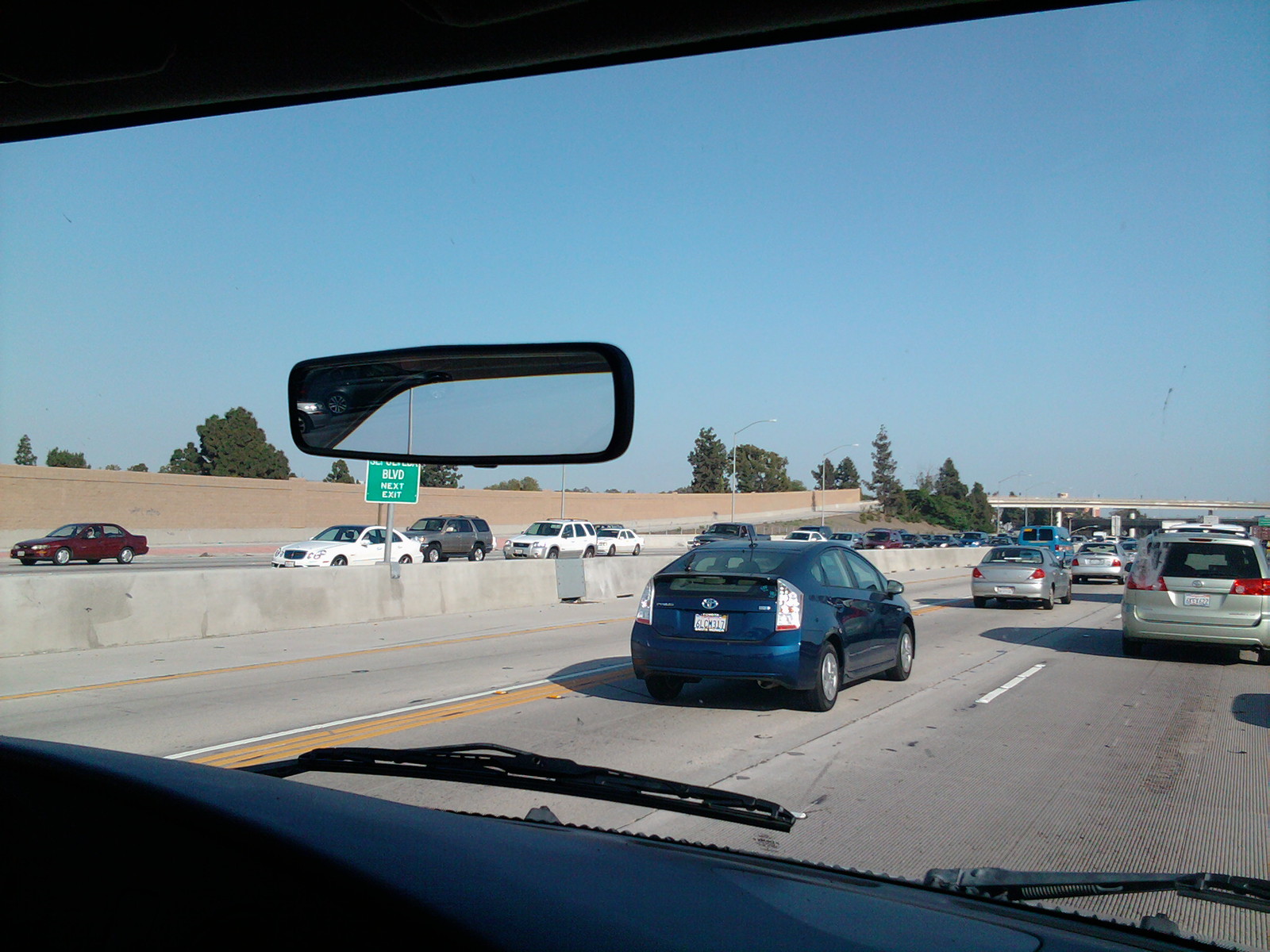The photograph captures a vibrant scene on an interstate highway during the daytime. The sky is a clear, brilliant blue, and a few trees are visible, adding to the picturesque setting. 

In the foreground, the interior of a car is partially visible, including the dashboard, rear-view mirror, and windshield with its wipers. The camera perspective is from the driver's seat, showing the car navigating the right-hand lane. Visible in the side mirror, multiple cars – at least twenty – populate the busy roadway.

Among the vehicles, a notable little blue hatchback with partly discernible numbers and letters on its rear license plate is situated on the far left. Numerous gray cars are also present, contributing to the bustling traffic flow.

A green road sign positioned on the median indicates the "Boulevard Next Exit," signaling an upcoming turn-off. In the distance, a bridge spans across the highway, under which the traffic continues to move smoothly. White lane markings divide the lanes, ensuring organized movement for the cars traveling in both directions.